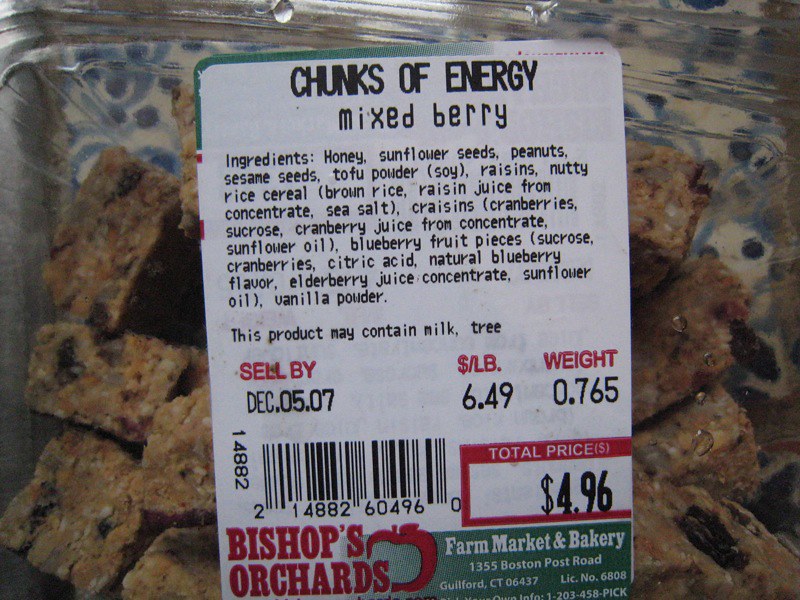The image features a photograph of a food product packaged in a clear plastic bag. The bag has a detailed label indicating the product name, "Chunks of Energy Mixed Berries," and contains small blocks of granola. The granola comprises honey, sunflower seeds, peanuts, sesame seeds, tofu powder, raisins, and nutty rice cereal, among other ingredients. The label also mentions a possible presence of milk and tree nuts.

The baggie rests on a table covered with a cloth that features white, blue, and light blue hues. Important product details include a "sell by" date of December 5th, 2007, and a total weight of 70.765 grams, priced at $6.49 per pound, making the total price $4.96. The label also includes a barcode.

At the bottom, the label reveals that the product is made by "Bishop's Orchards" written in bold red capital letters, accompanied by an apple logo. A green border beneath this states "Farm Market and Bakery," with the address, "1355 Boston Post Road, Guilford, Connecticut."

This thoughtfully composed product image captures the essence of the granola mix while also providing all relevant purchasing and manufacturing details.